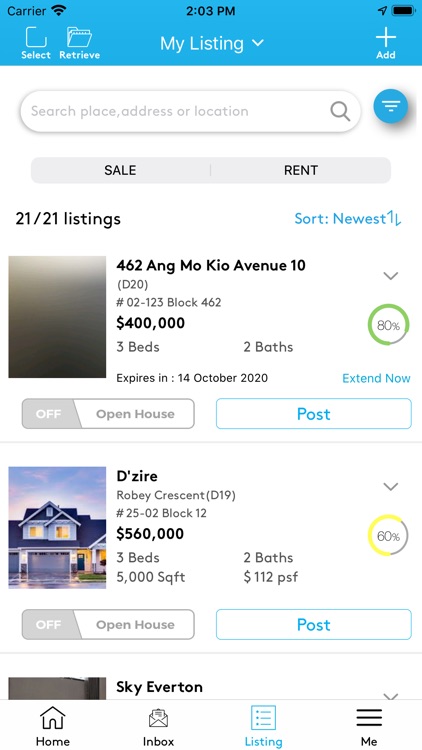This image is a screenshot taken from a smartphone displaying a housing listings application. 

At the top of the screen, the phone's carrier information is visible on the left side along with a black Wi-Fi icon. In the center of the top bar, the time reads 2:03 PM, and on the right side, a fully charged battery icon can be seen. The main application interface follows below this status bar.

Starting from the top section of the app interface, there's a blue banner that includes a "Carrier" label on the left, alongside a Wi-Fi icon, time in the center, and battery status on the right. Just underneath, the interface displays various options: "Select" and "Retrieve" with associated folder icons, and to the far right, there's an "Add" button represented by a plus sign.

Below this blue banner, the screen turns white, introducing a search bar which prompts the user to "search place, address, or location," with a blue tab menu icon situated to the right of the search bar. Directly beneath the search bar, there are two tabs labeled "Sale" and "Rent" for toggling between different types of housing listings.

The next section shows information about search results. On the left side, it indicates "21 of 21 listings," while on the right side, there's a filter option displaying "Sort by: Newest" in blue text.

Proceeding downward, the first housing listing is for "462 A&G Moquio Avenue, Unit 10," priced at $400,000 for a property consisting of 3 bedrooms and 2 bathrooms. Below this listing, users have the option to click "Post."

The second listing is titled "D'Zire" and is priced at $560,000. There is a front-view picture of the house on the left side, and text indicating the property features: 3 bedrooms, 2 bathrooms, spanning 5,000 square feet at $112 per square foot. There is also an option to post this listing.

The third listing only has the title "Sky Everton" visible. 

At the bottom of the screen, there are four navigation icons labeled "Home," "Inbox," "Listing," and "Me." 

Overall, the interface design facilitates easy browsing and management of property listings with clear, categorized sections and interactive options for users.